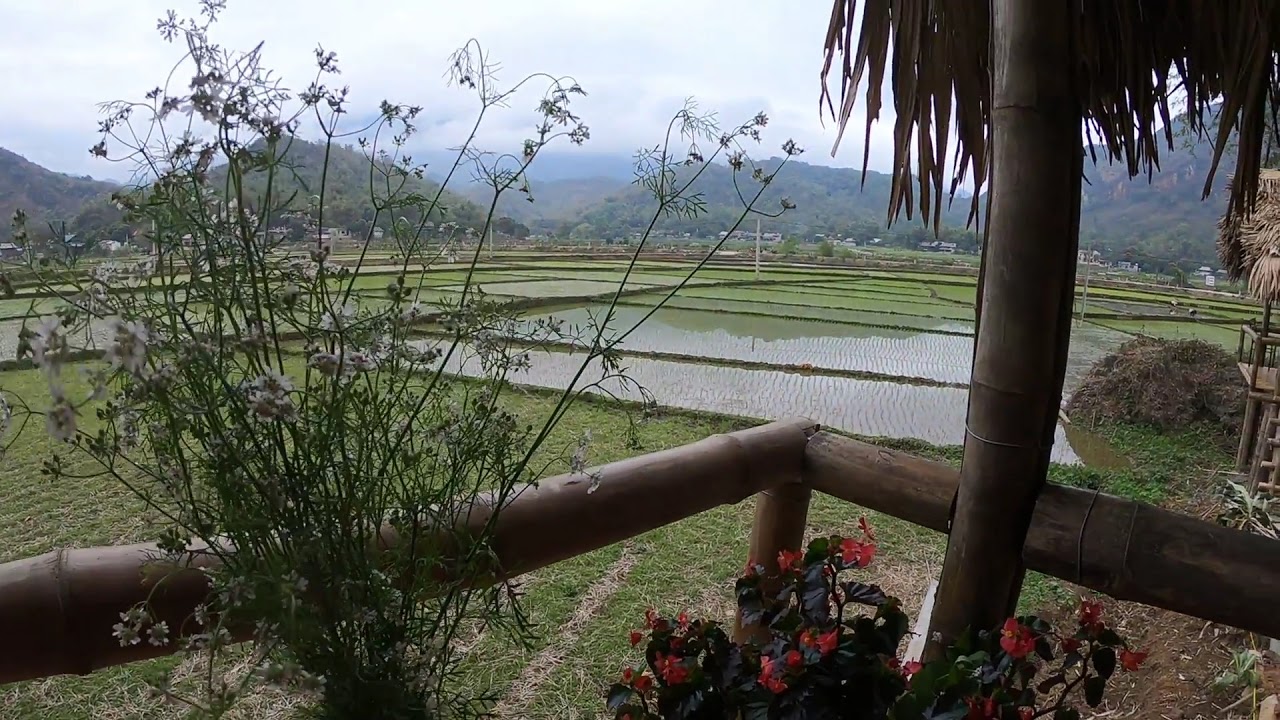The image captures a serene outdoor scene that appears to be a tropical agricultural area, possibly somewhere like Vietnam. Dominated by lush green hues, the background features rolling hills and mountain ranges densely covered in verdant trees under a somewhat cloudy sky. These hills slope down into a valley of rectangular agricultural fields, which might be rice paddies, interspersed with several lakes or flooded sections giving a grid-like appearance to the landscape. Closer to the foreground, a wooden fence-like barrier, resembling tree trunks fashioned into a railing, outlines a patio. Inside this barrier grows a palm tree and a scraggly bush adorned with blooming white flowers. The patio itself features a potted plant with dark leaves and red flowers, adding to the natural ambiance. Some huts with straw roofs and a pile of dirt are also visible, enhancing the rustic charm. Daylight bathes the scene, illuminating the expanse with soft light filtered through the mostly white clouds.